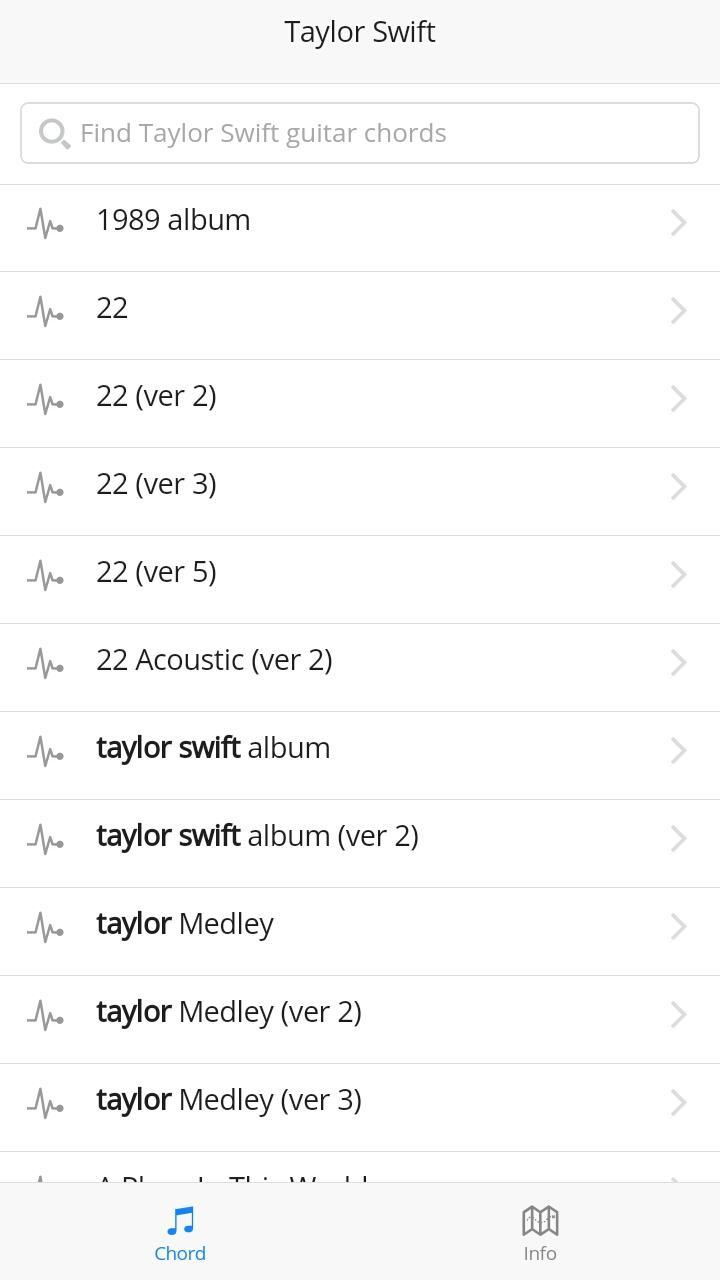The image showcases a phone search interface with a detailed Taylor Swift-related query. At the top, there's a light gray rectangle spanning the width of the screen, containing the black text "Taylor Swift." Immediately below, a white search bar with a light gray magnifying glass on the left prompts the user with "find Taylor Swift guitar chords."

Below the search bar, a list of search results is displayed in black text. The first entry reads "1989 album" with a right-pointing directional arrow next to it. Subsequent results include various versions of the song "22," each accompanied by a right-pointing arrow: "22" followed by "22 (version 2)," "22 (version 3)," "22 (version 5)," and "22 (acoustic version 2)."

Further down, the search results list different Taylor Swift albums and medleys, each with versions indicated in parentheses and arrows pointing to the right: "Taylor Swift album," "Taylor Swift album (version 2)," "Taylor Medley," "Taylor Medley (version 2)," and "Taylor Medley (version 3)."

At the bottom of the image, there are options labeled "Chord" on the left and "Info" on the right. The detailed layout suggests the user is looking for specific guitar chord variations and details related to Taylor Swift's music.